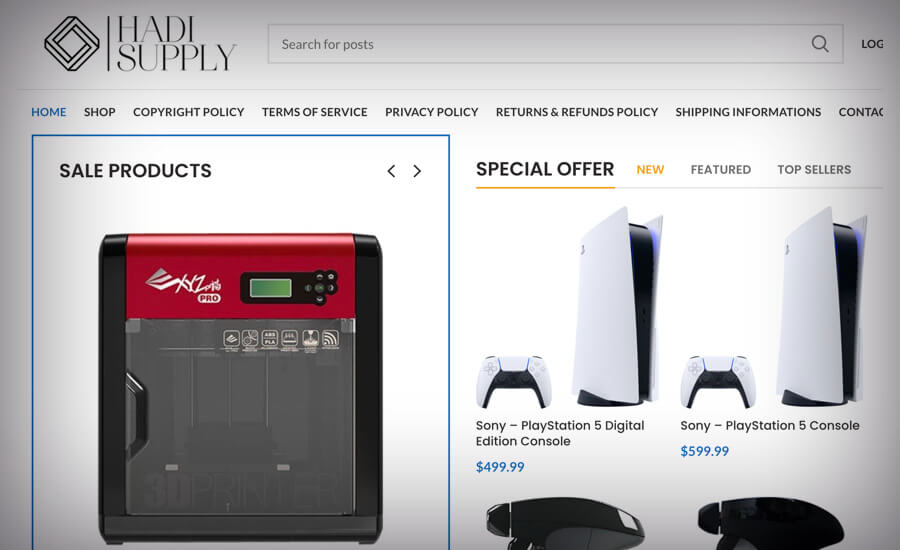The image depicts a photograph of a computer screen displaying a portion of a website. The photograph is framed with noticeable shadows at the top and bottom edges, confirming that it is indeed a photo of the screen rather than a screenshot.

At the top of the webpage, there is a black diamond-shaped logo with a vertical line through it, followed by the text "Haddie Supply." Below the logo, a search bar invites users to "Search for posts," with a login option positioned to the right.

Directly beneath the header, a navigation menu displays several options: "Home" (highlighted in blue), "Shop," "Copyright Control," "Terms of Service," "Privacy Policy," "Returns and Refunds Policy," "Shipping Information," and "Conact" (notably missing the 'T').

Further down the page, a product display area features a blue-outlined rectangle with curved corners. This section is labeled "Sale Products" and includes navigational arrows for browsing back and forward. The focal product appears to be a metallic box with a red panel on top, adorned with small white text, a tiny green LED indicator, and a grey bottom portion.

To the right of this product display, a sidebar contains several headings: "Special Offer," "New," "Featured," and "Top Sellers." The "Special Offer" heading is underlined in yellow. Below this section, two white objects resembling PlayStation controllers are displayed.

The left controller is labeled "Sony PlayStation 5 Digital Edition Console" and priced at $499.99. The right controller, labeled "Sony PlayStation 5 Console," is priced at $599.99. The bottom of the photograph reveals just the tops of two curved black objects, whose full forms are not visible.